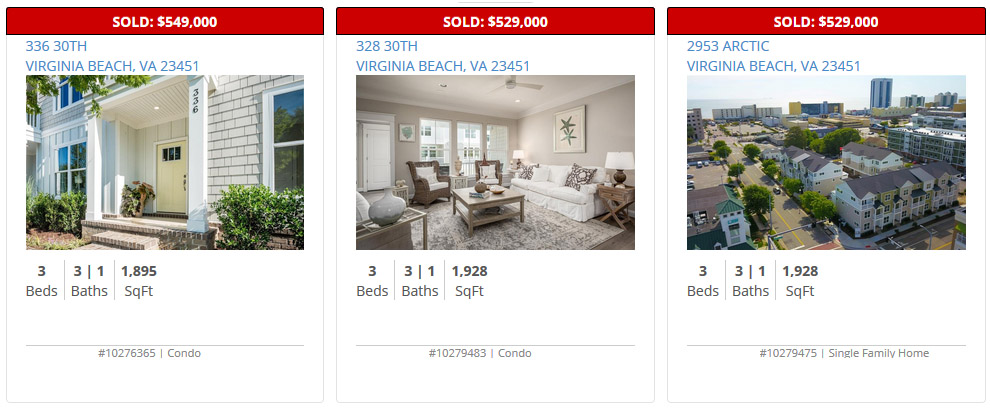Three recently sold properties are highlighted at the top with red bars showcasing the sale prices: $549,000, $529,000, and $529,000. Below the prices, there is blue text listing the addresses of the properties:

1. 336 30th Street, Virginia Beach, VA 23451
2. 328 30th Street, Virginia Beach, VA 23451
3. 2953 Arctic Avenue, Virginia Beach, VA 23451

Beneath the addresses, there are images of the respective homes. The first image depicts a traditional Southern-style home with columns and a brick facade. The second image shows the interior of a living room furnished with couches, chairs, tables, and paintings. The third image provides a bird's eye view of one of the properties.

Each property features three bedrooms and three and a half bathrooms. The first property has a living space of 1,895 square feet, while the second and third properties each have 1,928 square feet.

Finally, beneath these images and descriptions, additional details classify the properties: two are condos, and one is a single-family home.